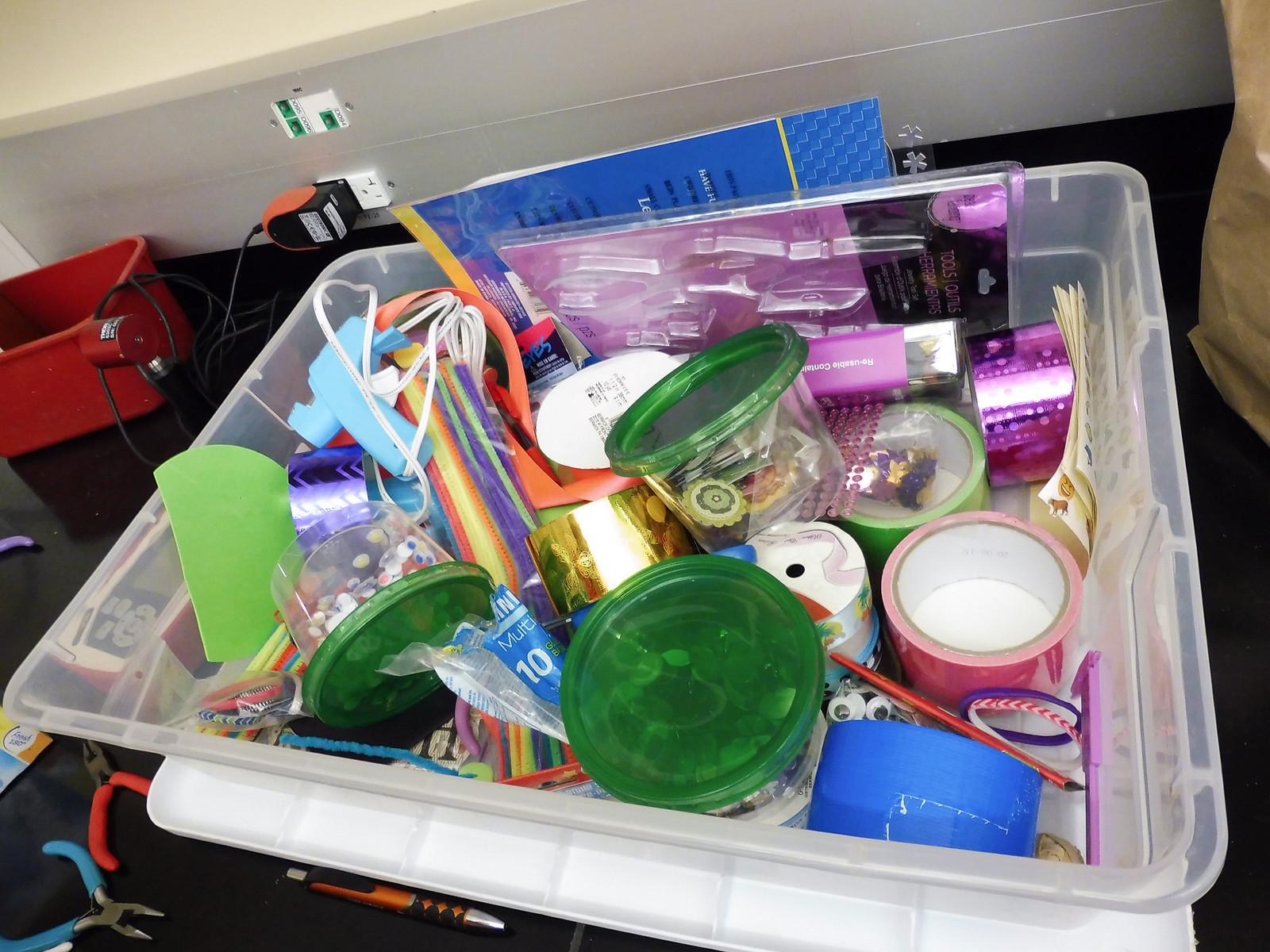A vibrant photograph captures a clear plastic storage bin brimming with an array of colorful crafting materials. The contents of the bin are organized in smaller clear plastic containers, each adorned with brightly colored lids, predominantly green, that house a delightful assortment of stickers, beads, googly eyes, and buttons. Various rolls of colored duct tape, including hues of blue, hot pink, and green, are neatly arranged within the bin, adding to the rainbow of artistry supplies. A radiant collection of pipe cleaners in shades of purple, green, yellow, and red extend their long tendrils, promising endless creation possibilities. Additionally, the bin contains clear plastic bags and housing containers that appear designed for scissors, though the scissors themselves are absent, indicated only by their silhouettes impressed on the plastic. Sheets of paper covered with diverse animal stickers add to the collage of crafting potential. This entire assortment is positioned on the floor, surrounded by an assortment of tools, depicting a creative workstation ready for imaginative endeavors.